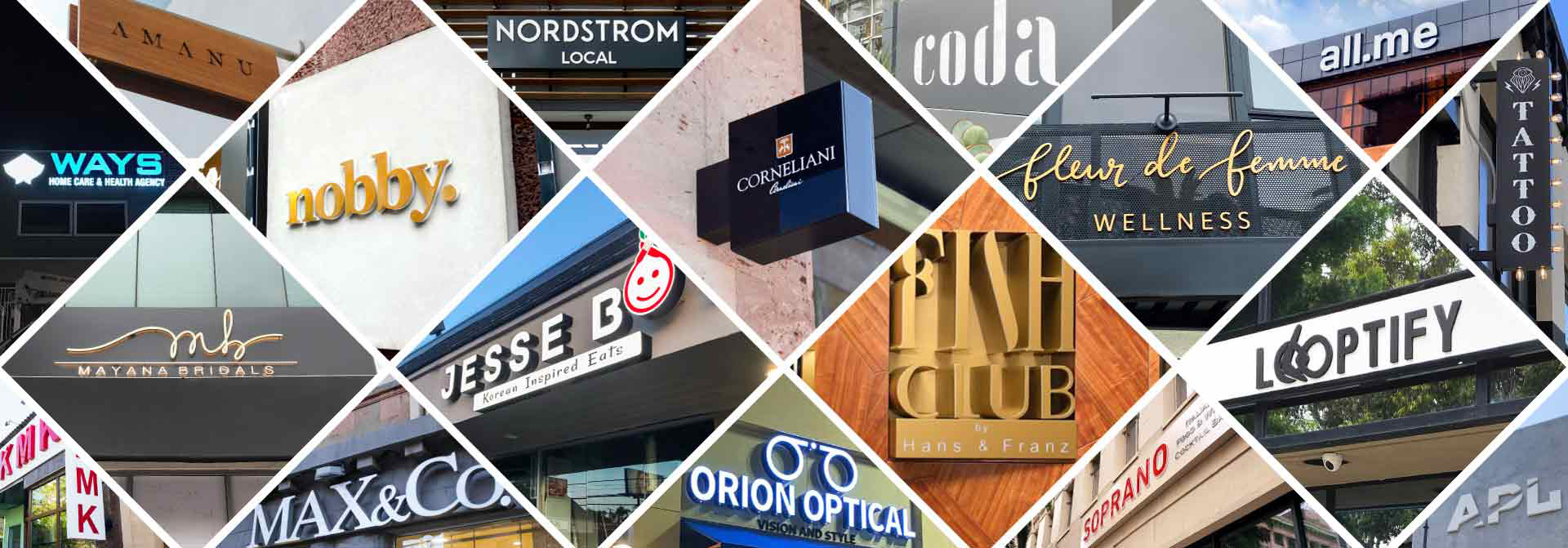The image showcases a wide rectangular collage of interconnected diamond and triangular storefront signs, each delineated by distinct white borders. The storefronts, either half or full diamonds, represent a variety of brands including Knobby, Nordstrom Local, Coda, All.Me, Looptify, Orion Optical, Fish Club, Max and Company, Waves, Soprano, APL, and Tattoo. Noteworthy details include Knobby's gold letters, Nordstrom Local's black backdrop, Jessie B accompanied by a smiley face, and Fish Club displayed on a wooden background with gold lettering. Additionally, Fleur de Femme Wellness features a black sign, and Orion Optical is marked by a neon pair of glasses.